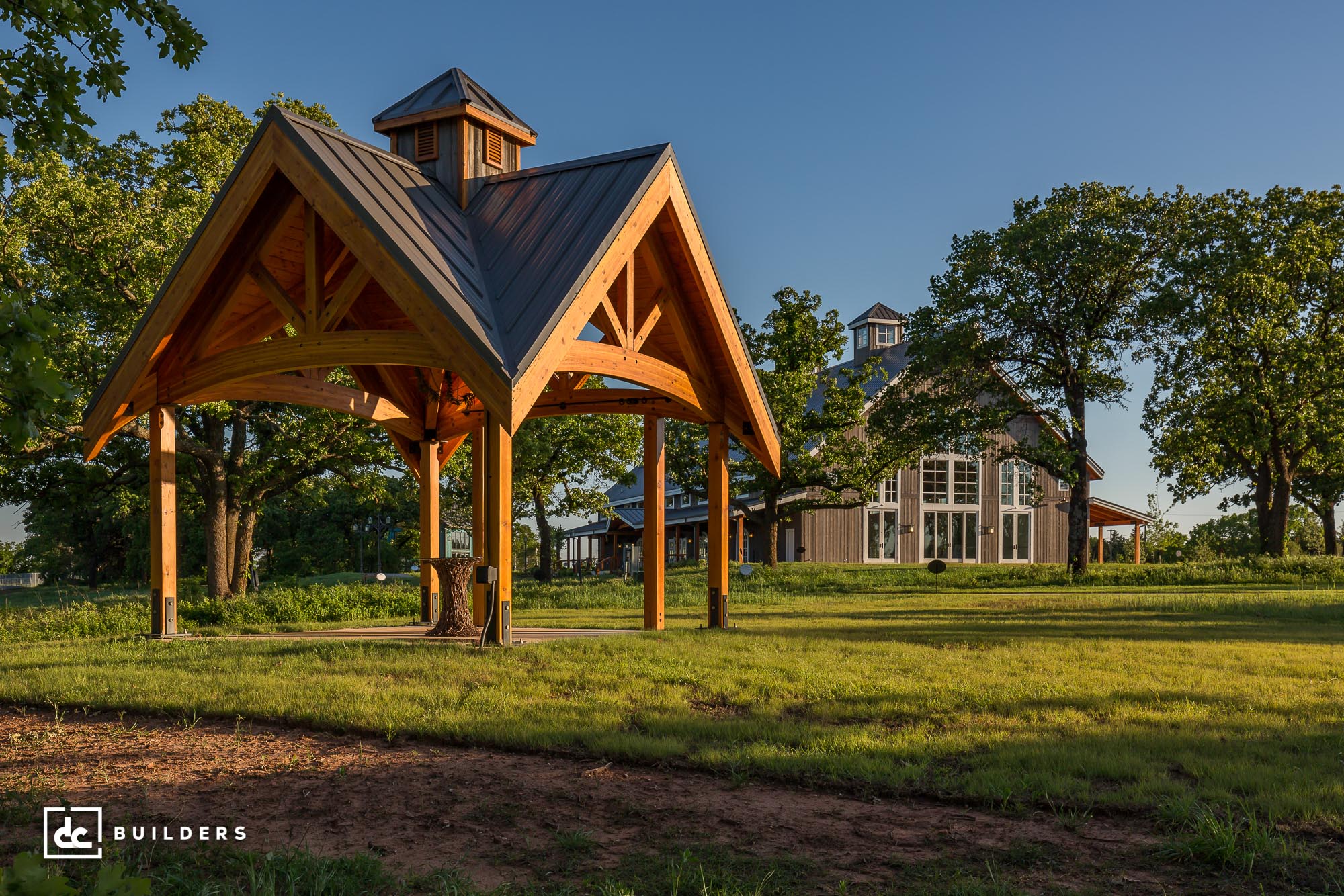The image depicts a beautifully handcrafted wooden gazebo set in a lush field of green grass, surrounded by trees. The gazebo features six tall, natural wood posts and a dark gray metal gabled roof with a triangular shape at each corner, crowned by a cupola. In the center of the gazebo, there appears to be a tree trunk used as a seat and a small table resting on a concrete pad. The backdrop reveals a large, gray barn-style house with a similar cupola on its roof. This impressive structure boasts high ceilings, expansive white-framed windows, and white French doors, giving it a grand mansion-like appearance. The house includes a front porch with an awning and roof overhangs on both ends. The sky overhead is clear and blue, adding to the serene and picturesque setting.